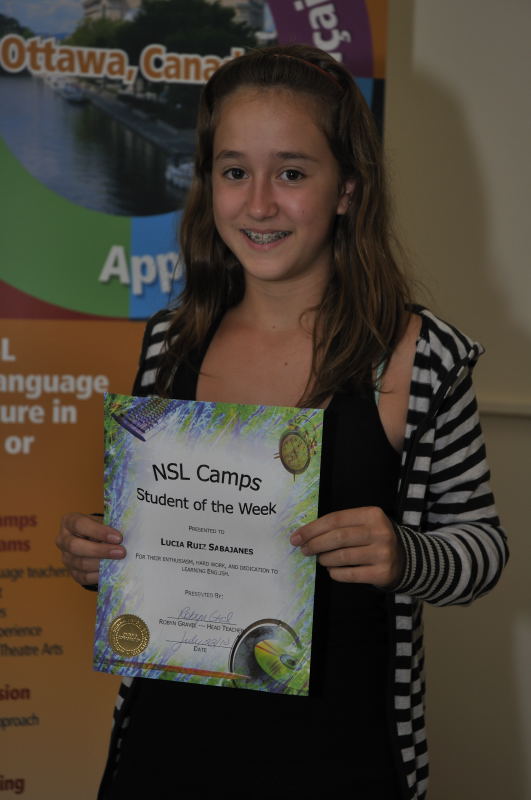This image features a smiling middle school-aged girl named Lucia Ruiz Sabah Yanis, proudly holding a colorful certificate titled "NSL Camps Student of the Week," awarded for her enthusiasm, hard work, and dedication to learning English. Lucia has long brown hair adorned with a red thin headband, braces, and is looking directly at the camera. She is wearing a black tank top or dress beneath a black and white striped sweatshirt. The certificate she holds has vibrant blue and green borders with designs depicting a keyboard, a clock, and CDs, and includes a gold seal in the lower left corner. In the background, there is a partially visible banner that reads "Ottawa Canada," suggesting the camp is located in Canada. The background wall appears to be off-white, contributing to the organized and celebratory atmosphere of the photo.